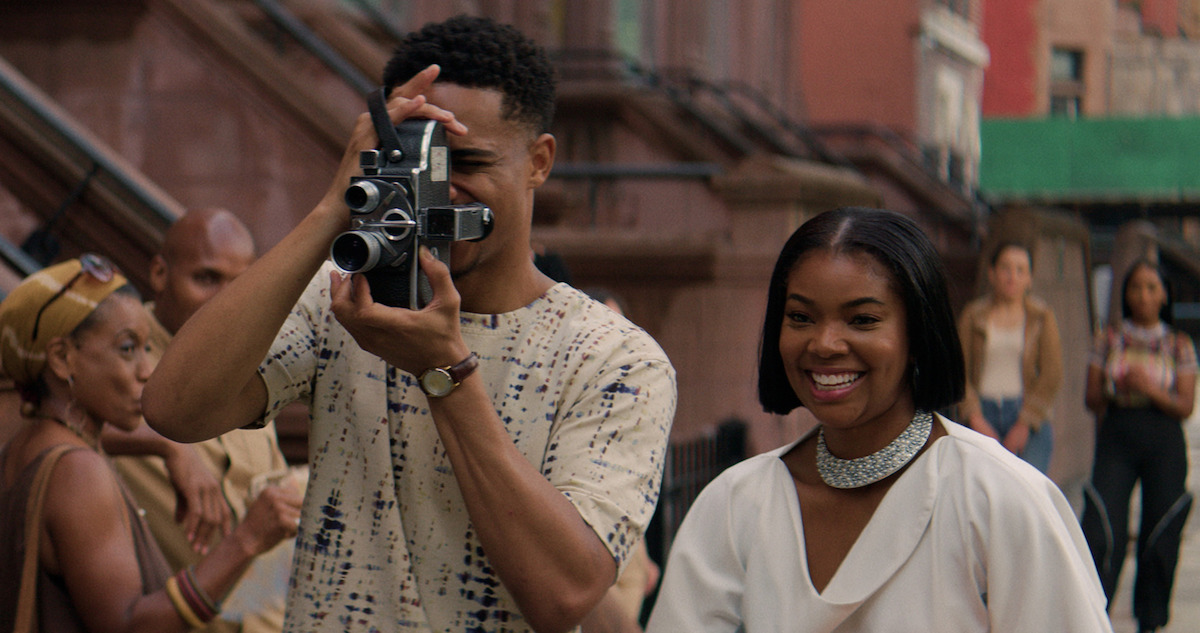A bustling city street is depicted with a large building prominently in the background, featuring red brick and numerous windows. In front of one building, there's a small green canopy. The sidewalk is crowded with pedestrians. Among them, a young Black man holding a movie camera is filming something ahead of him. He wears a white shirt with black print. Beside him, a young Black woman in a white dress adorned with a light-colored, likely silver necklace, stands. Her beautiful black hair contrasts against her attire. The scene captures the lively urban atmosphere with people moving around the two central figures.